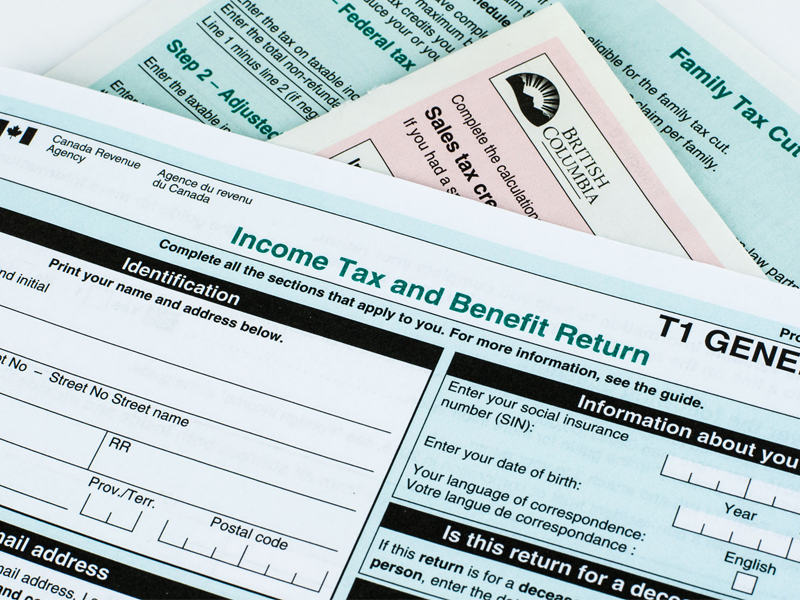The image displays three stacked income tax papers against a light gray background, visible only in the top corners. The papers, arranged diagonally and taking up nearly the entire frame, consist of multiple layers with detailed text for tax-related information. The top document prominently features the text "Canada Revenue Agency" and "Income Tax and Benefit Return" with a mix of green border and green background sections. It includes numerous fields for personal information such as name, address, social insurance number, and date of birth, along with directives to complete applicable sections for tax returns. Beneath it, a pink and white document labeled "British Columbia" with a sun logo, partially visible, contains phrases like "complete the calculation" and "sales tax." The third document, seen in the upper right corner, bears the title "Family Tax Cut" and, like the others, has multiple blank lines for entering personal and financial details. The overall setting suggests a legal or administrative task, likely the process of sorting or filing taxes.